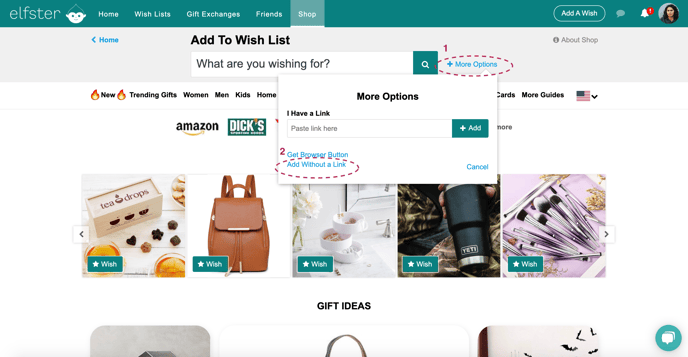This detailed screenshot of the Elfster website showcases its interface and features prominently. At the top of the page, a green navigation bar stretches across the screen with the Elfster logo on the far left side. Adjacent to the logo is an icon depicting an elf's head, characterized by green hair and a simple white face with two eyes, a nose, and a smile.

The navigation bar houses several menus: Home, Wishlist, Gift Exchanges, Friends, and Shop. Directly below this, because the Shop section is selected, you see a search bar and the title "Add to Wishlist." To the left is the option to return home, while to the right is a "More Options" button, which is highlighted by a red dotted circle and labeled as number one. Activating this More Options button opens a white pop-up box with the heading "More Options." Within this box, there's a bar labeled "I have a link" next to it is a green "Add" button featuring a plus sign.

Beneath this More Options box, another option is marked with a red label number two which states "Get Browser Button or Add Without a Link," with "Add Without a Link" also highlighted by red dotted lines. Below this, the rest of the webpage displays images of various products available to add to a wishlist, such as tea drops, a brown backpack, a bathroom organizer, a Yeti mug, and makeup brushes. These items are categorized under a title menu that includes sections like new, trending gifts, women, men, kids, and more.